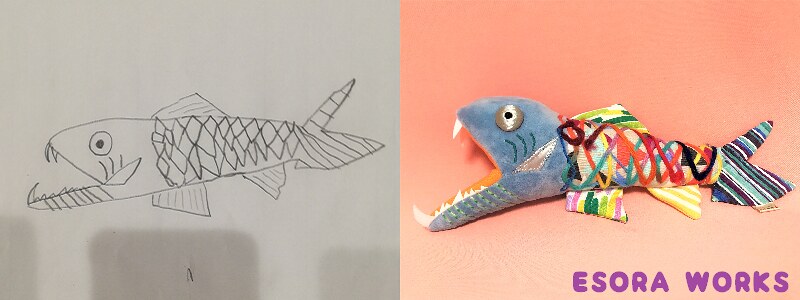This image features a side-by-side comparison of a child's drawing and its plush toy counterpart. On the left, a pencil sketch depicts a whimsical and slightly menacing deep-sea fish, with exaggerated features that evoke both cuteness and a hint of terror. The backdrop is formed by three rectangular shadows, possibly from foams. The sketch is monochromatic, rendered in shades of white and charcoal gray. 

On the right, the imaginative drawing has been transformed into a colorful stuffed animal. The plush fish faithfully mirrors the child’s creation but is now vibrantly blue with rainbow accents. Its mouth, wide open, reveals sharp, protruding teeth, adding a playful touch to its ferocious design. The background here is peach-colored, and at the bottom it features the text "Isora Works" in purple, likely indicating the company responsible for bringing this delightful creation to life.